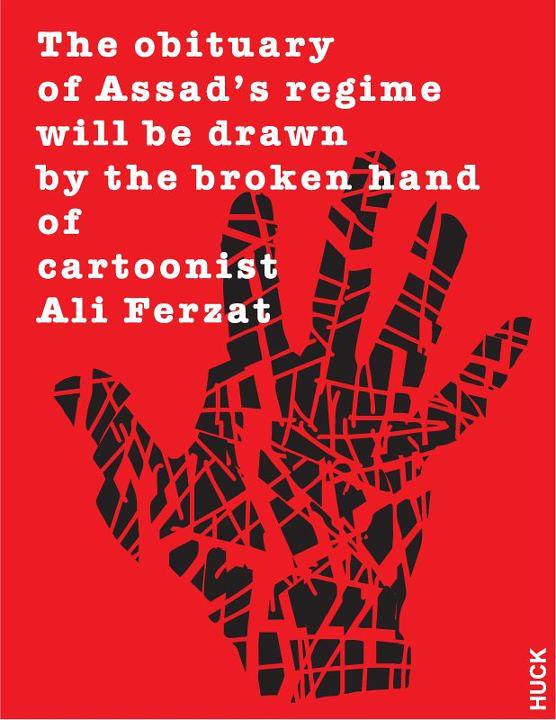The image features a vivid red background, dominated by an artistic graphic of a hand occupying nearly half of the visual space. The hand, which is clearly illustrated rather than realistic, is painted black with white stripes forming a crisscross pattern, creating an impression of fragmentation. In the lower right-hand corner, a small segment of the hand is emblazoned with the word "Hawk" in vertical letters, ascending slightly from the bottom. An accompanying caption in white, typographic font reads, "The obituary of Assad's regime will be drawn by the broken hand of cartoonist Ali Farzat," with only the initial letters of key words capitalized.